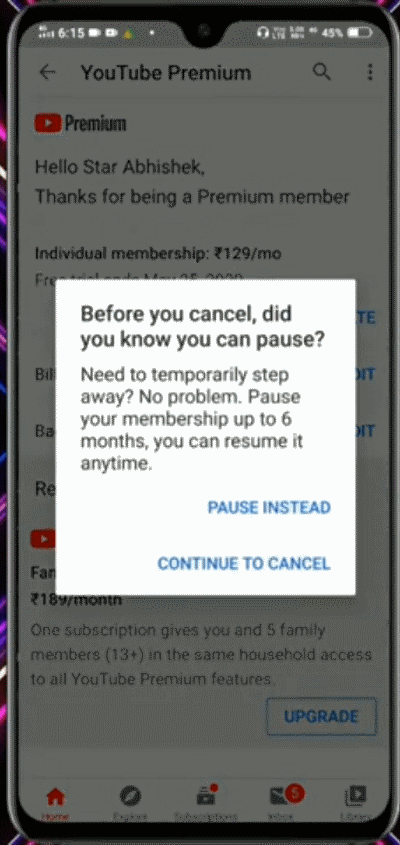The image is a screenshot taken from a mobile phone, featuring a black border. At the top, there is a thin light gray line displaying the current time, which reads 6:15. To the right of the time, the phone's battery icon indicates a 45% charge. 

Below this top section, there is an arrow pointing left next to the text "YouTube Premium," accompanied by the YouTube logo, which is a white box with a red play button inside it. The text "Premium" appears adjacent to the logo. Further down, a personalized message reads: "Hello star ABHISHEK. Thanks for being a Premium member."

Beneath the greeting, there is an overview of available memberships, specifically highlighting an "Individual membership" priced at $129 per month.

Centrally located within the screenshot is a white pop-up box with black text, which overlays the membership details. The pop-up reads: "Before you cancel, did you know you can pause? Need to temporarily step away? No problem. Pause your membership up to six months. You can resume at any time." 

At the bottom of the white box, in blue text, there is an option stating, "Pause instead," followed by another option below it in standard text reading, "Continue to cancel."